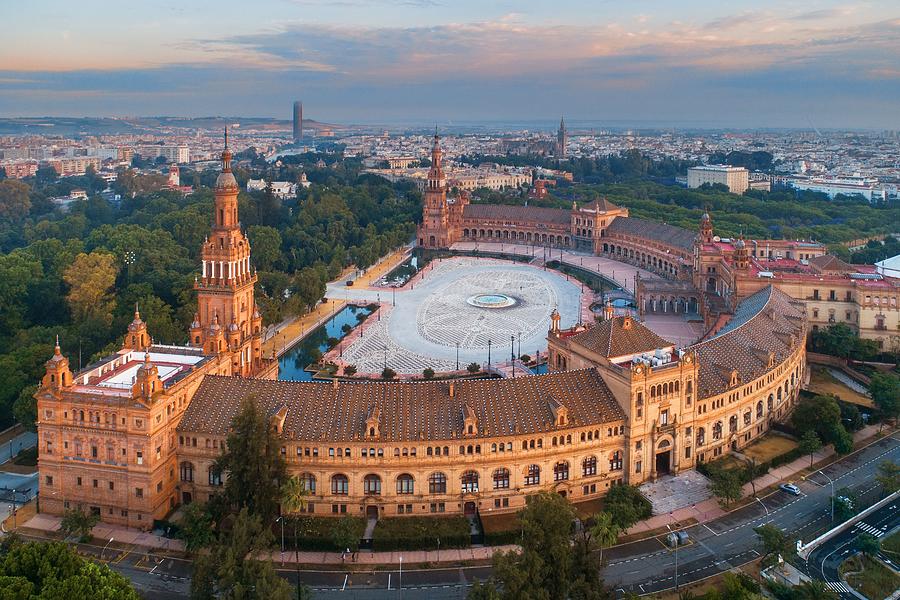This horizontal rectangular image depicts an ornate, semi-circular building constructed from yellow-tan stone, featuring many arched windows and brown rooftops. The building is shaped like a 'D' or an arc, with a prominent square structure and a tower at the left end, reminiscent of a church. The building surrounds a central area containing a gray stone-paved surface and a fountain, encircled by green and yellow bushes and trees, as well as streetlights. 

The scene is set in an urban environment, with numerous other buildings, primarily white or tan, visible in the background under a mostly cloudy sky with hints of blue and patches of blue and pink-hued clouds. The horizon reveals tall buildings jutting into the sky. 

In the foreground, a gray street outlined with white and yellow dashed and solid lines curves along the front of the building, accompanied by additional streets to the right corner. Surrounding the building is a mix of green bushes and trees, with a gray sidewalk and a tan pavement area enhancing the scene.